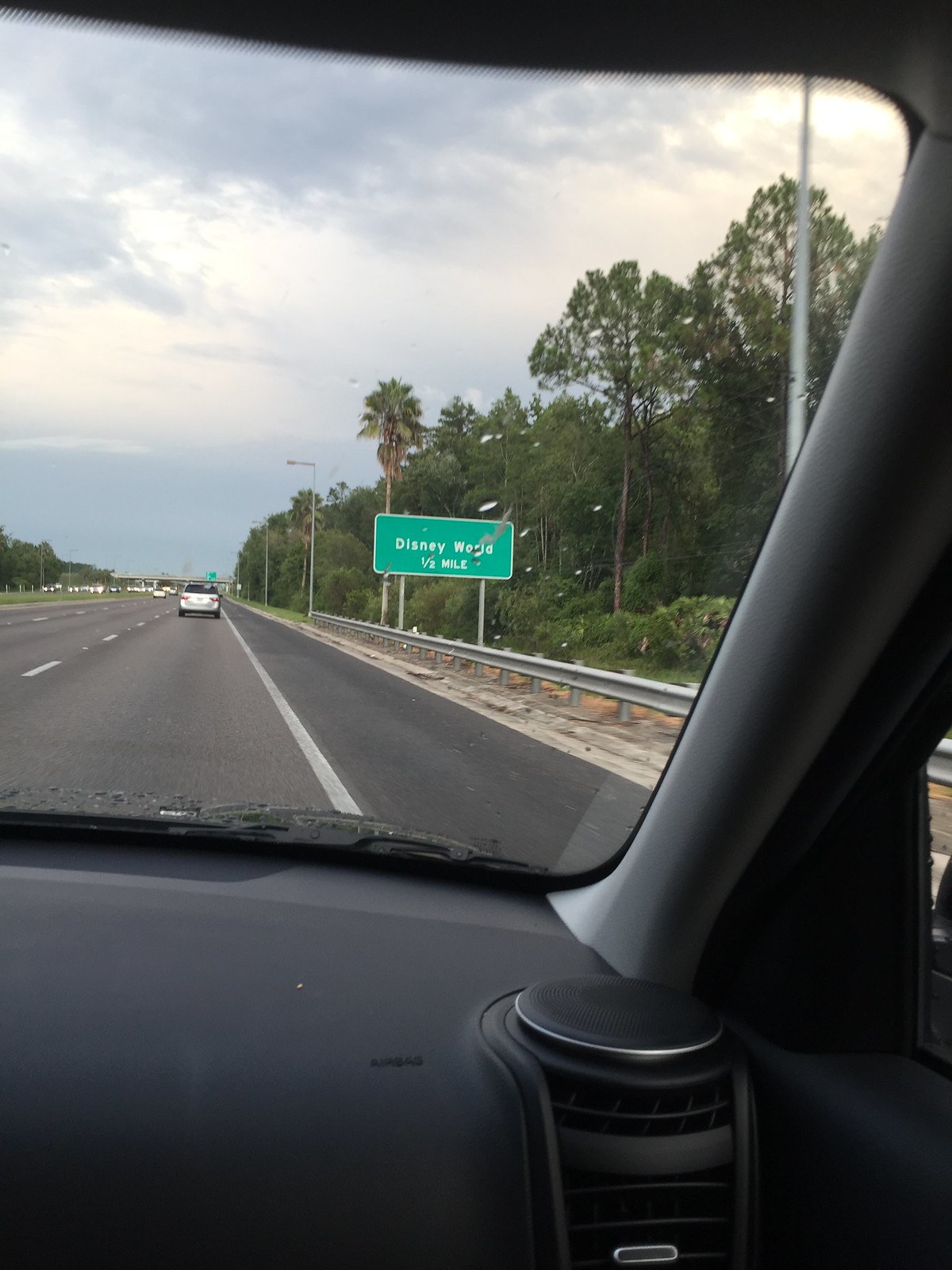This detailed image is a color photograph taken from the passenger seat of a vehicle, capturing an open highway scene in Florida. Through the windshield, one can see an overcast sky with some sun peeking through the clouds in the top right corner. The car cruises in the far right lane of a three-lane freeway, demarcated by white dashed lines and a solid line on the right edge. Directly ahead, a silver minivan leads the way. On the right side of the image, a prominent green highway sign supported by two silvery posts announces "Disney World: 1/2 Mile." The scene is embellished with street lamps and power lines extending from the ground on the right side, just before the center divider. The roadside features a mix of green bushes and trees, including several palm trees, emphasizing the Floridian locale. The grass appears lush, with some sandy dirt patches visible. The interior of the car reveals a black dashboard and a glimpse of an AC vent in the bottom right corner. A silvery guard rail runs parallel to the road, adding to the structured elements of this highway setting.